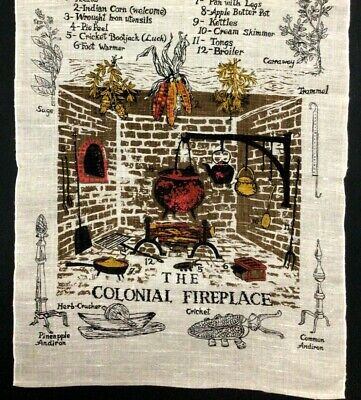This is a detailed photograph of a vintage linen tea towel titled "The Colonial Fireplace." The central image, rich in historical ambiance, vividly depicts a classic colonial fireplace centerpiece with bricks, a large black iron armed bar, and various cooking implements. Prominently, a reddish copper kettle and a copper skillet with yellow cornbread hang over the fire from the iron bar, which also supports additional cooking tools. The lower hearth area holds a skillet and other undefined items, perhaps used for cooking.

Herbs and bunches of Indian corn are intricately illustrated drying above the mantle, adding an authentic rustic charm. The fireplace bricks reveal subtle earthy tones, with the main bricks in brown and some areas showing red. Surrounding the colorful central illustration are black and white drawings detailing various colonial-era items like a foot warmer and a large wooden bread bowl with a roller.

Additionally, the white cloth of the tea towel, mounted on a black backboard, features inscriptions around the periphery. These are not recipes but explanations of the items depicted, such as "Indian corn for welcome," "apple butter," "kettles," "a broiler," and more, giving context to the historical artifacts. The combination of color and detailed drawings against the linen fabric presents a vivid narrative of a colonial kitchen, making it a collectible item for enthusiasts of vintage linens and historical depictions.